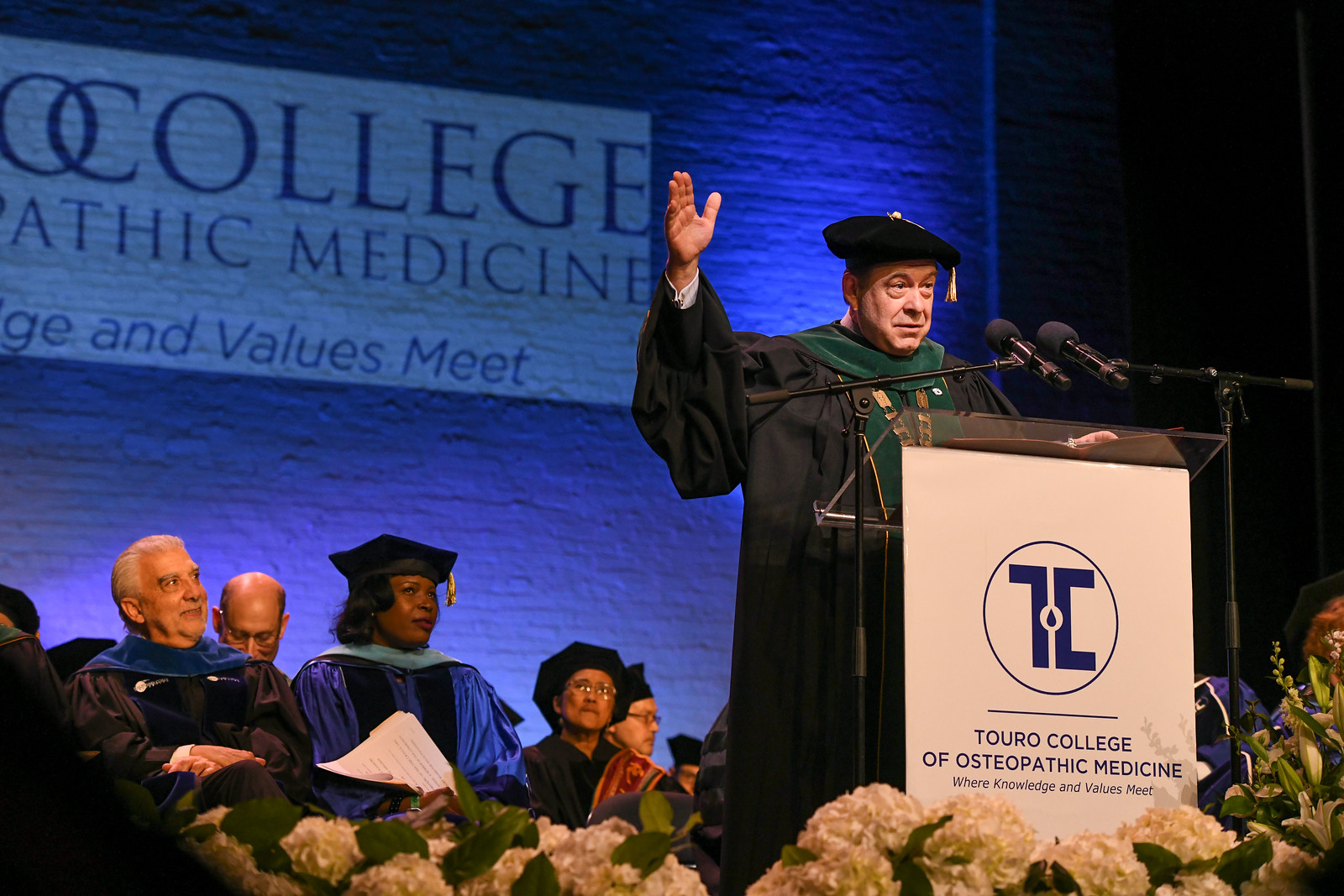In the image, a man stands at a podium giving a speech during what appears to be a graduation ceremony for Touro College of Osteopathic Medicine. He is dressed in black robes, a black cap, and a green scarf, with his right hand raised in a gesture. The podium, which features a logo consisting of a "7" and a "C" with a teardrop in between, bears the text "Touro College of Osteopathic Medicine" and the slogan "Where Knowledge and Values Meet." In front of the podium, there are white flowers with green leaves.

Behind him, seven individuals are visible, most of them wearing black caps and gowns. A black woman is seated in the center, holding a piece of paper, flanked by a mix of men and possibly women. The background features a projected image on a brick wall, reiterating "Touro College of Osteopathic Medicine" along with the partially visible slogan "where knowledge and values meet," illuminated by blue lighting.